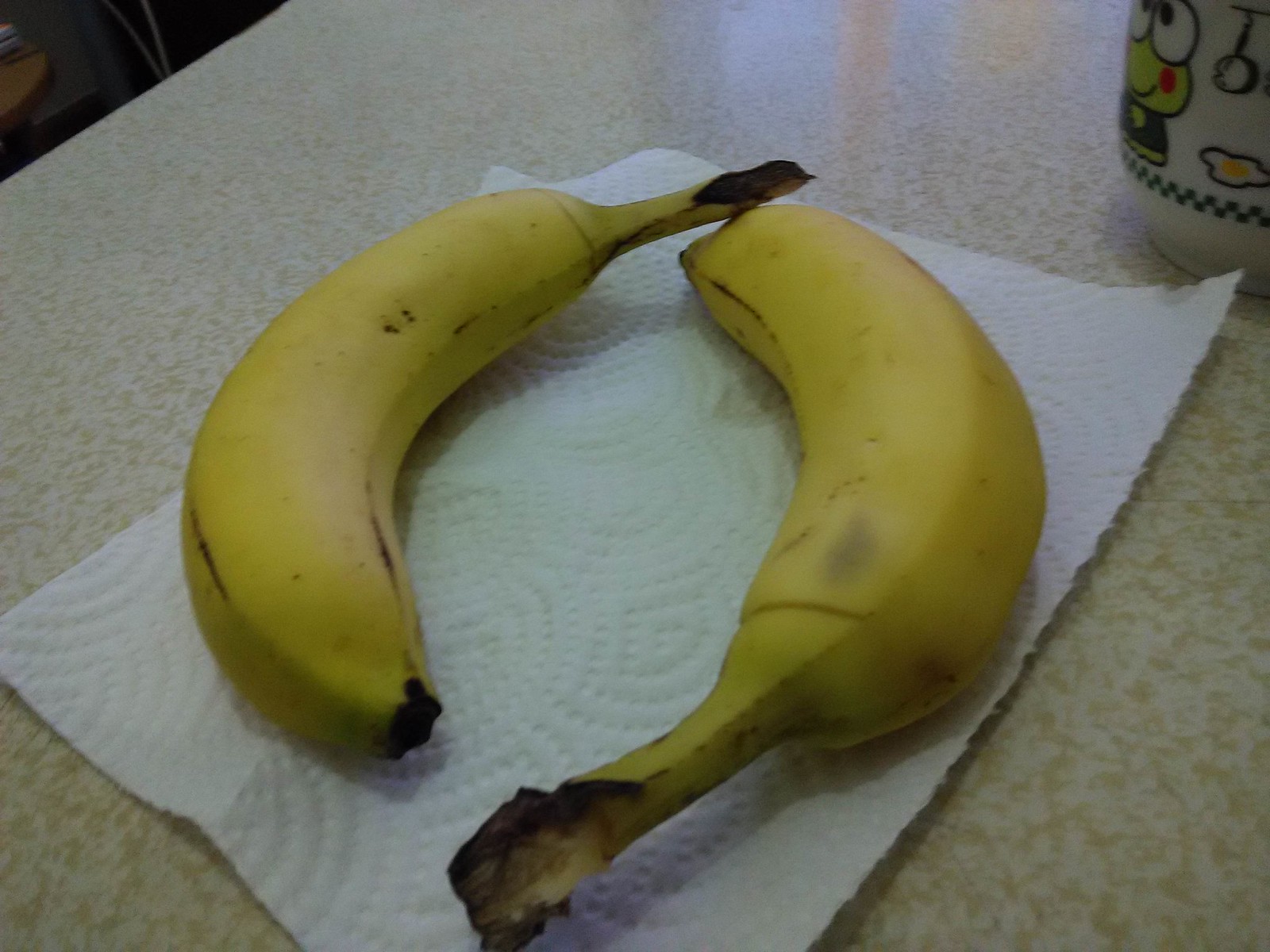In this photo, two yellow bananas with subtle touches of brown and green, indicating near-ripe status, rest on a sheet of white kitchen roll adorned with concentric shell patterns. The bananas are positioned opposite each other, creating a circular, "zero" shape—one with the stalk at the top and the other with the stalk at the bottom. They lie atop a countertop with a marble effect surface, suggesting a kitchen setting. In the top right corner, a white ceramic mug is partially visible. The mug features a simple green illustration of a frog and a fried egg motif beside it, adding a whimsical touch to the scene.